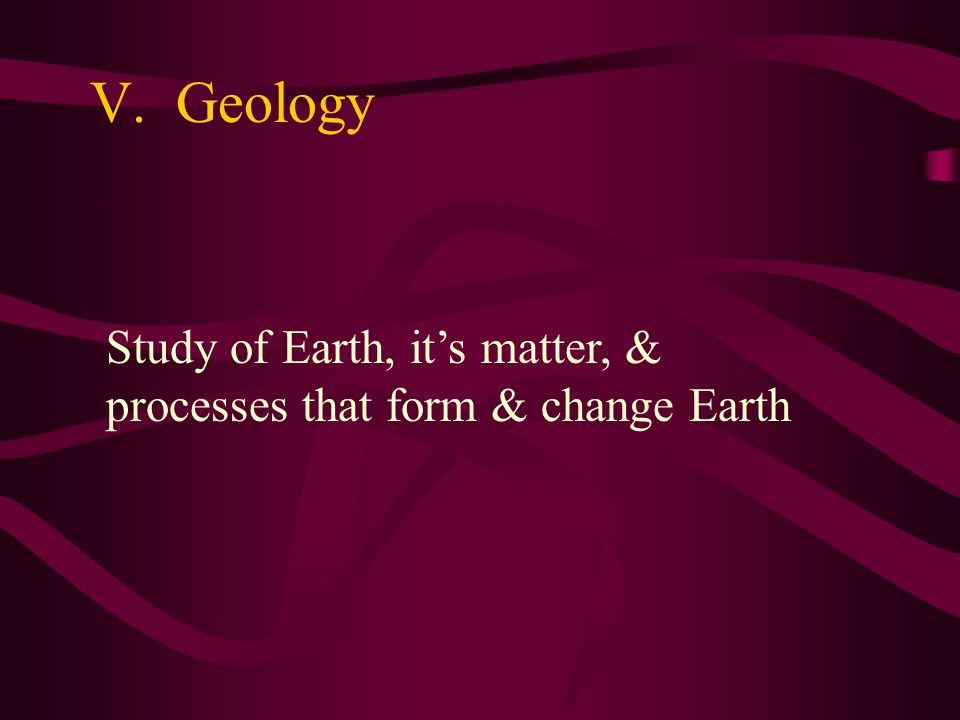This image appears to be a slide or cover from a digital textbook or flashcards, characterized by a burgundy background adorned with wavy, ribbon-like stripes in varying shades of burgundy. In the top left corner, there's a yellow-colored text displaying "V. Geology," where the "V" indicates a chapter number or section, and "Geology" is written in a matching yellow font. Prominently centered in white font is the definition of geology: "Study of Earth, its matter, and processes that form and change Earth." The overall design features about four to five stylish ribbons across the background, contributing to a visually appealing layout with blackish edges.